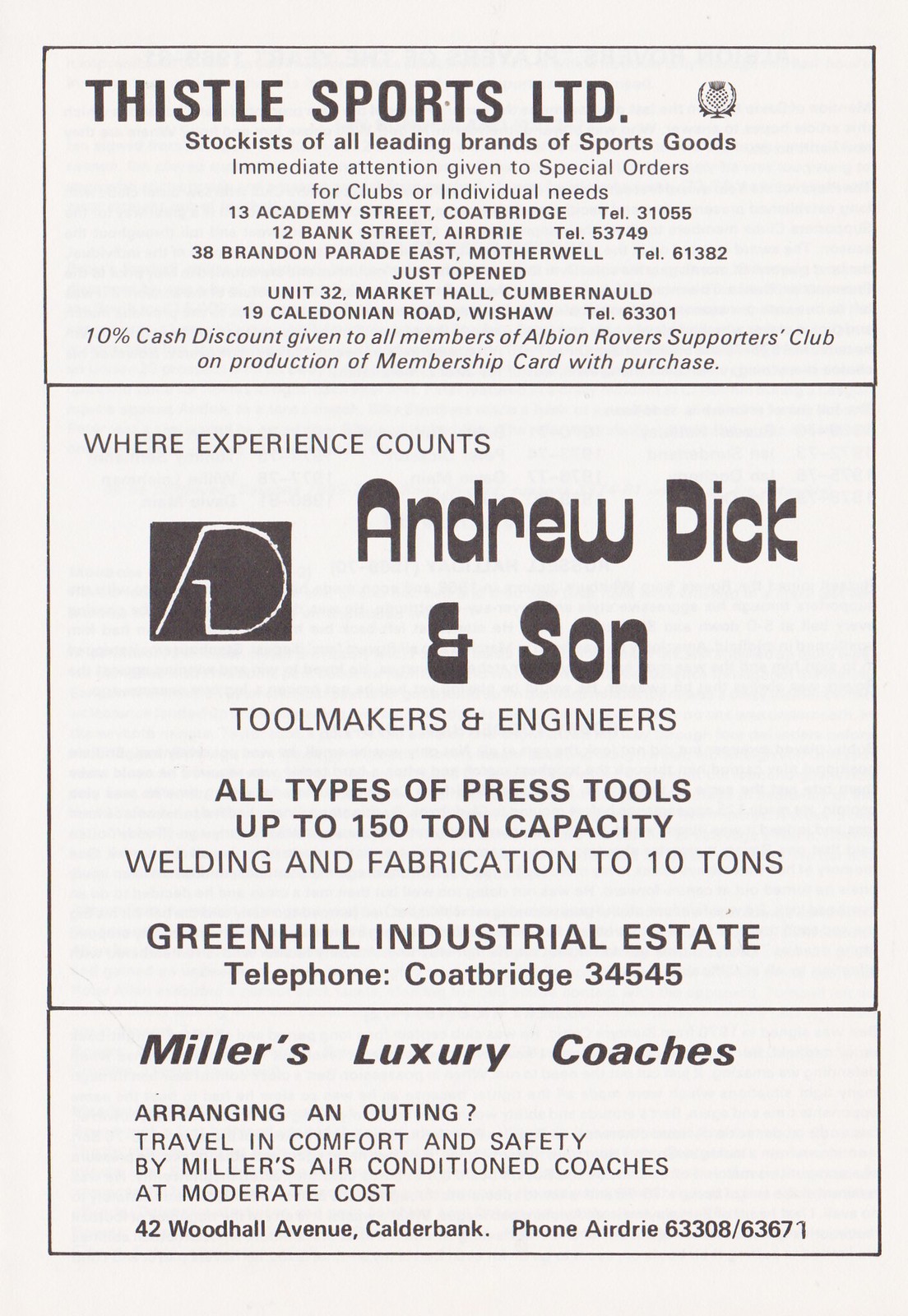This image is a rectangular advertisement listing, likely from a newspaper or a match day magazine. It consists of three ads, each framed with a thin black line on a white background, featuring black print. 

The top ad is for Thistle Sports Limited, which stocks all leading brands of sports goods. It highlights that special orders for clubs or personal needs receive immediate attention. The ad lists several addresses: 13 Academy Street, Coatbridge (Tel: 31055), 12 Bank Street, Airdrie (Tel: 53749), 38 Brandon Parade East, Motherwell (Tel: 61382), Unit 32 Market Hall, Cumbernauld, and 19 Caledonian Road, Wishaw (Tel: 63301). A 10% cash discount is offered to members of the Albion Rovers Supporters Club upon presenting a membership card.

The middle ad focuses on Andrew Dick & Son, toolmakers and engineers. It boasts of considerable expertise with press tools up to 150-ton capacity, as well as welding and fabrication work up to 10 tons. The business is located in Green Hill Industrial Estate, and the given telephone number is Coatbridge 34545.

The bottom ad promotes Miller’s Luxury Coaches, emphasizing comfortable and safe travel arrangements facilitated by their air-conditioned coaches at a moderate cost. The contact information provided is 42 Woodhall Avenue, Bank; the phone number is Airdrie 63308 or 63671.